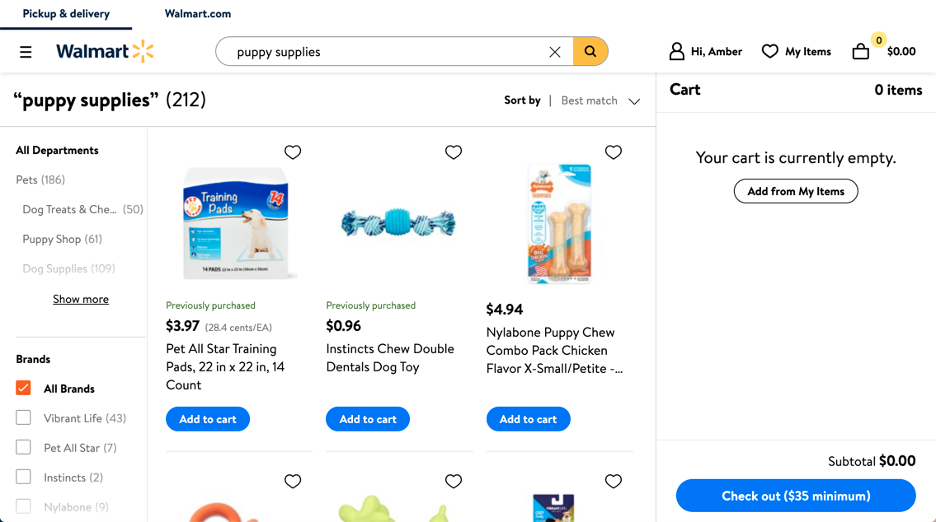This image is a screenshot from the Walmart website, specifically the online store section for "puppy supplies." At the top of the page, it indicates that 212 items match the search term "puppy supplies," which is displayed both in quotes and parentheses (212). The upper-right corner of the webpage shows the account information belonging to a user named Amber, with a greeting "Hi, Amber" displayed next to the user icon. Below this, the shopping cart icon, which features a yellow circle indicating its status, shows that the cart is currently empty with a "0" and "0.00" (zero dollars).

Beneath Amber's account details, there is a notification section for "My Items" and an empty cart summary stating, "Your cart is currently empty." The minimum amount for checkout is also noted as $35. The user appears to have clicked on the "All Brands" filter, as evidenced by the three items displayed per row on the page. Among the listed items, you can see a variety of puppy supplies, including a chew toy and puppy pet training pads.

The overall layout is clean and organized, providing clear information about the user's account details, their shopping cart status, and the available puppy supplies.